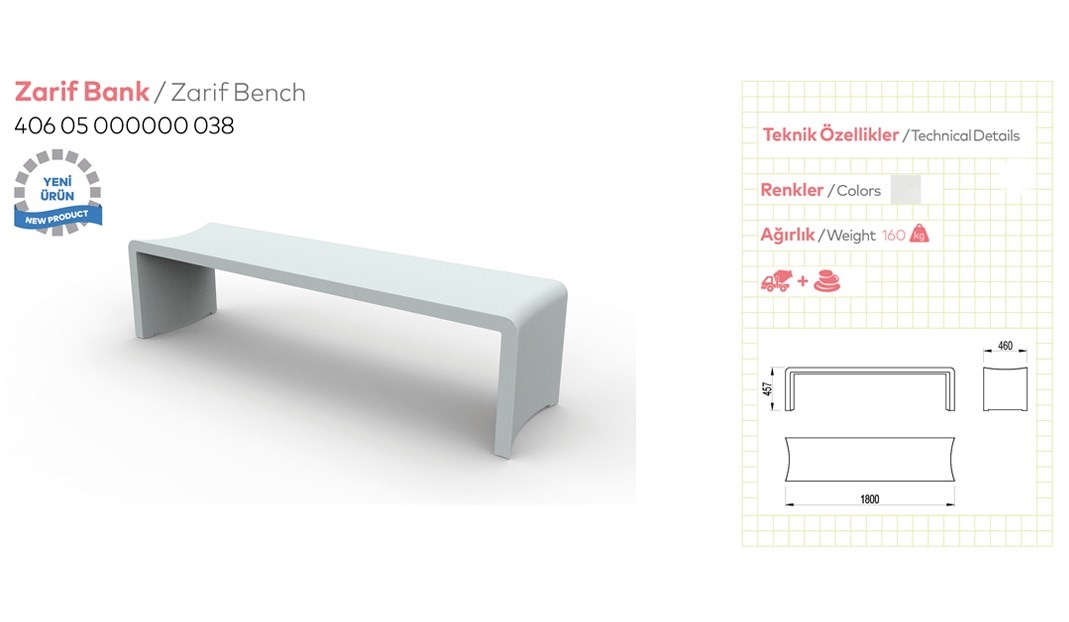The image features a white background. On the left side, there is a rendered graphic of a sleek, minimalistic bench with two legs at either end, resembling a plank with its ends bent downwards, all in white. Above this rendering, the text "Zerif Bank" appears in red, followed by "Zerif Bench" in gray and underneath in black text, it states the number 406050000038. On the right side, against a white background with a yellow grid, a detailed schematic of the bench is provided. This schematic includes sections in both English and another language, specifying "Technik Ozyklikr/Technical details," "Wrinkler/Colors" labeled as white, and "Agrylik/Weight" listed as 160 kg. The dimensions are clearly noted as 475 mm high, 460 mm wide, and 1800 mm long. Additionally, there are illustrations of a cement truck and stones, accompanied by the text “Yeni Ürün/New Product.”